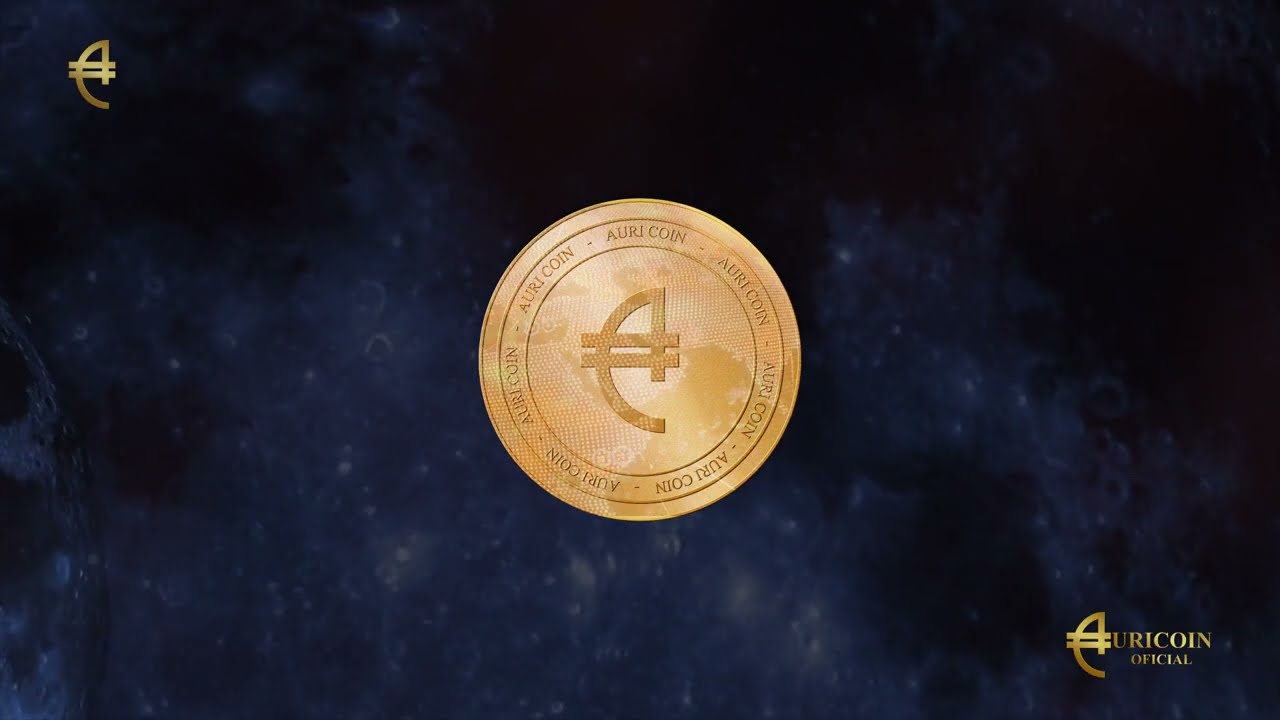The digital image features a gold coin prominently centered against a dark blue, ethereal background that resembles outer space, complete with twinkling stars and stardust accents. The gold coin bears a distinct symbol in its center, with the word "AURICOIN" repeatedly inscribed around its smooth outer rim. The emblem is designed to rise up straight before swooping down into a half-circle with two lines crossing at the top. This same emblem appears in the upper left corner of the image. In the bottom right corner, the image reads "Auricoin Official" beside the same emblem. The background's blotchy, dark navy hue, interspersed with white splotches, enhances the celestial theme of the image.